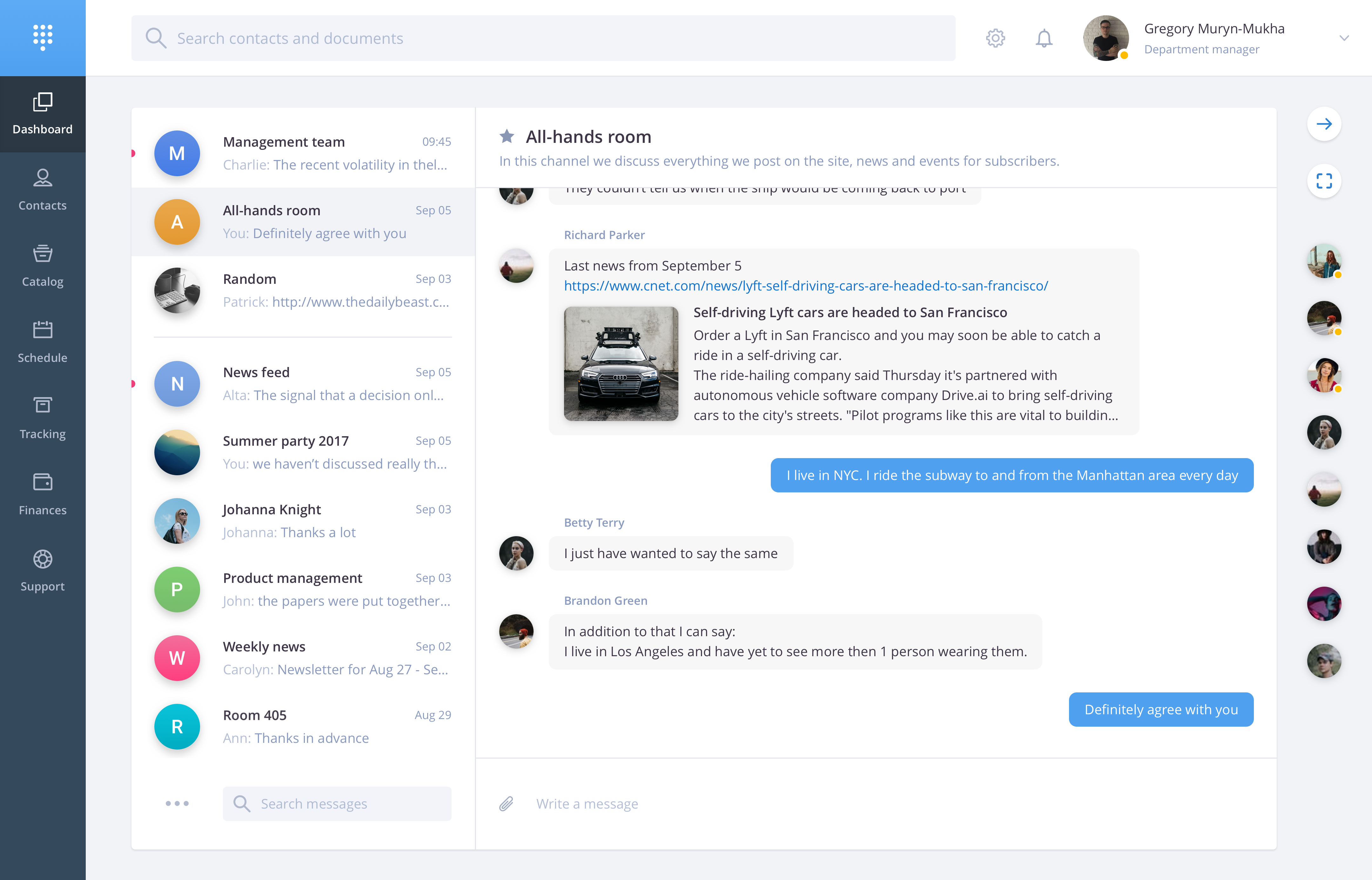The image is a horizontally rectangular screen capture of a messaging app interface. On the far left is a vertical navigation bar with a light blue top background fading into a darker bluish-black background. The menu items listed vertically from top to bottom are: Dashboard, Contacts, Catalog, Schedule, Tracking, Finances, and Support. 

At the top of the frame, running horizontally, there is a search bar labeled "Search Contacts and Documents." To the right of this bar are three icons: the Settings icon, the Notification icon, and an Avatar. Next to the Avatar, the name "Gregory Murenmuka" (spelled M-U-R-Y-N dash M-U-K-H-A) is displayed, along with the title "Department Manager."

The remainder of the screen is divided into two sections. On the left, there is a list of contacts and chat rooms, including: Management Team, All Hands Room (which is highlighted), Random, News Feed, Summer Party 2017, Johanna Knight, Product Management, Weekly News, and Room 405.

On the right side, the detailed view of the "All Hands Room" chat is displayed, revealing a text messaging thread within that specific room.